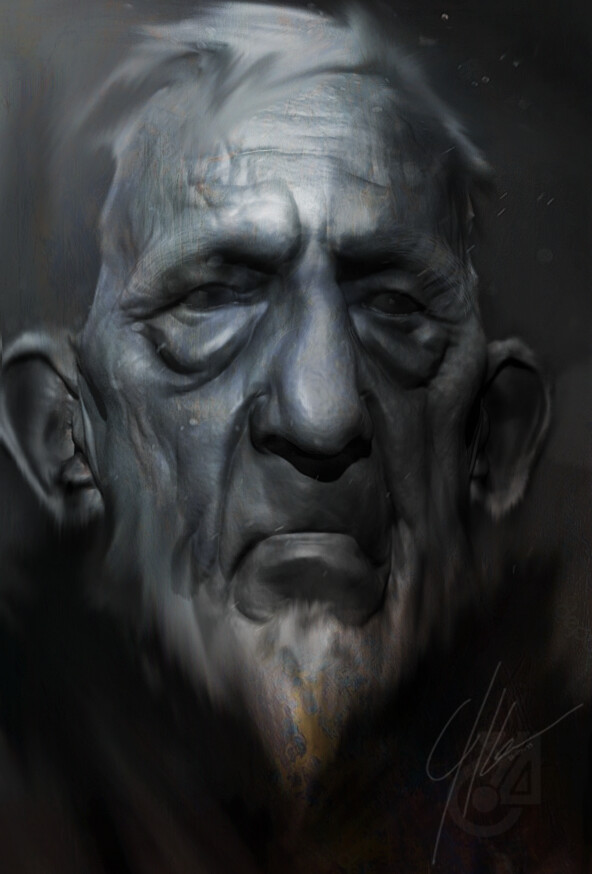This digital illustration depicts a very old man with a deeply wrinkled, pear-shaped face and pronounced bags under his eyes. His hair is wispy and white, predominantly on the top of his head, while the sides appear sparse. The man's facial hair includes a wispy white beard on his chin, notably without a mustache. His forehead features distinct wrinkles and a gold-accented mole. The image, rendered primarily in shades of black, white, and gray, includes subtle gold touches on the beard and forehead, and possibly hints of red. The man's eyes are sunken, with puffy areas above his left eyebrow, and his large nose and fine, pressed lips add to his weathered appearance. His face is slightly tilted away from the camera yet remains centered in the composition. The background is plain, with a barely discernible signature in the bottom right corner, and a watermark containing letters, possibly "Y," "A," and "O" with a bullseye motif. There are hints of robes that the man might be wearing, contributing to the artistic and old photo-like quality of the image.